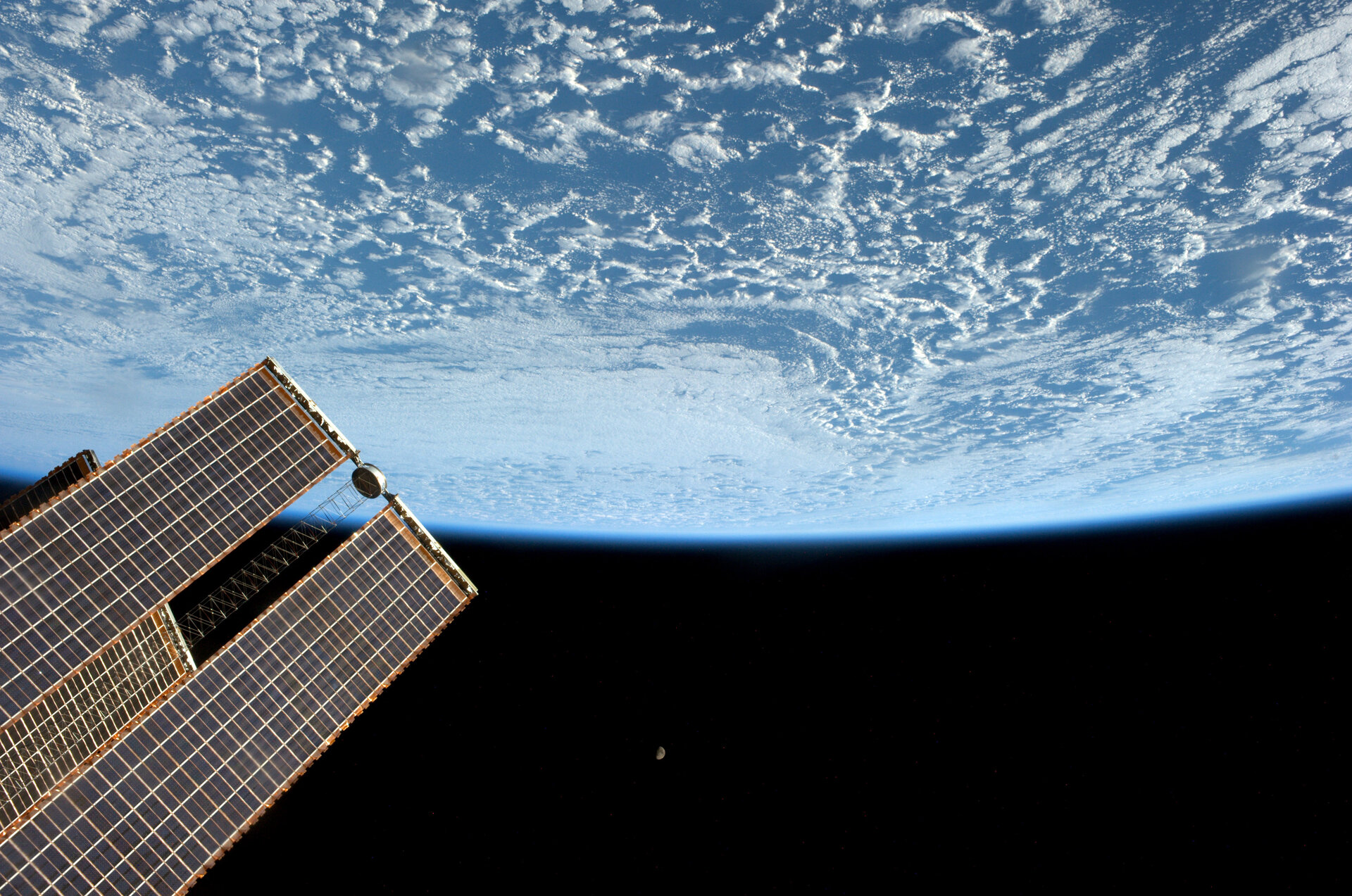This photograph, captured from a satellite in space, predominantly displays our planet Earth occupying the upper half of the image. Earth's surface is adorned with visible clouds, which give it the appearance of having snowy peaks amidst vast stretches of blue ocean. The bottom half of the image is dominated by the dark, starless void of outer space. In the bottom left corner, a satellite is visible, featuring blue solar panels with white pattern lines forming small squares; it has three sections, with the left and right panels being the same size and the middle section slightly smaller and thinner. Near the bottom center of the image, there is a small, distant gray object, likely the moon, subtly blending into the darkness of space. The image is devoid of any text, presenting a clear and uninterrupted view of this striking scene from space.